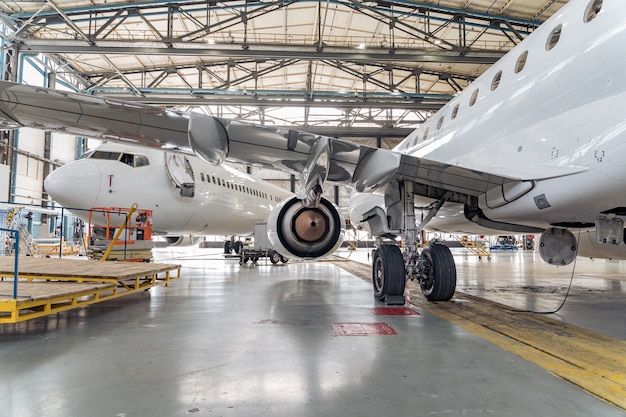This detailed indoor photograph captures the expansive interior of a large airplane hangar. Inside this massive facility with gray concrete floors, you can see two primarily white airplanes. The closer airplane on the right side of the image prominently displays its landing wheels resting on yellow lines painted on the floor, with blocks placed under the wheels to prevent rolling. You can also observe one of its engines, which features a copper-colored center, and a thin tube or electrical cord connected to it. This airplane's front wheels and one wing are visible, along with several of its windows. The second airplane is positioned farther back on the left, with its front end angled towards the left middle of the frame and its back end facing the center. Scattered around are various pieces of equipment and pallets, although their specific details are not clear. The overall impression is one of an industrial space dedicated to airplane maintenance or assembly.